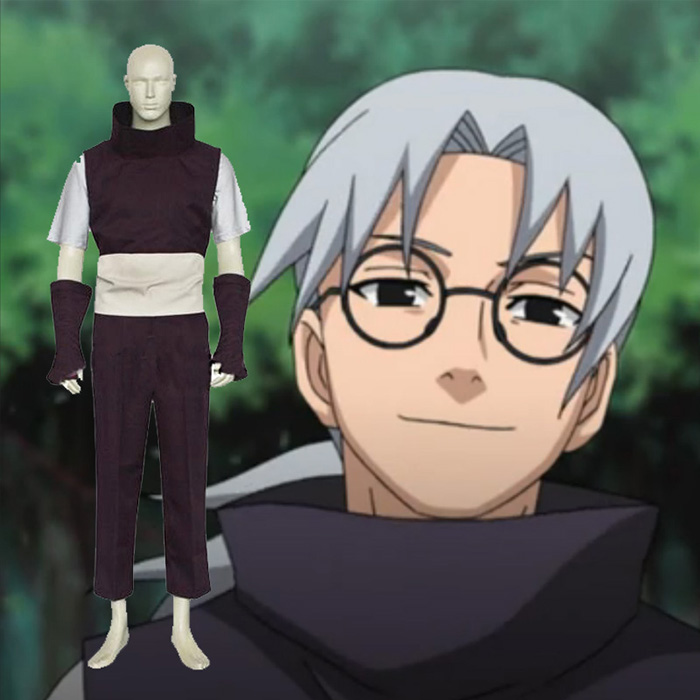The promotional image showcases a costume inspired by a Japanese anime character. On the left side of the image, a white male mannequin displays the costume, which consists of black pants that end just above the ankles, a white sash around the waist, and a black shirt with an exceptionally high, loose collar and short gray sleeves. The mannequin also wears black fingerless gloves that extend up to the elbows. In the background, partially visible, is the anime character the costume is based on. The character has gray hair, black glasses, and a prominent tall black collared shirt. The depicted scene provides a detailed comparison between the mannequin showcasing the elaborate costume and the original animated character.